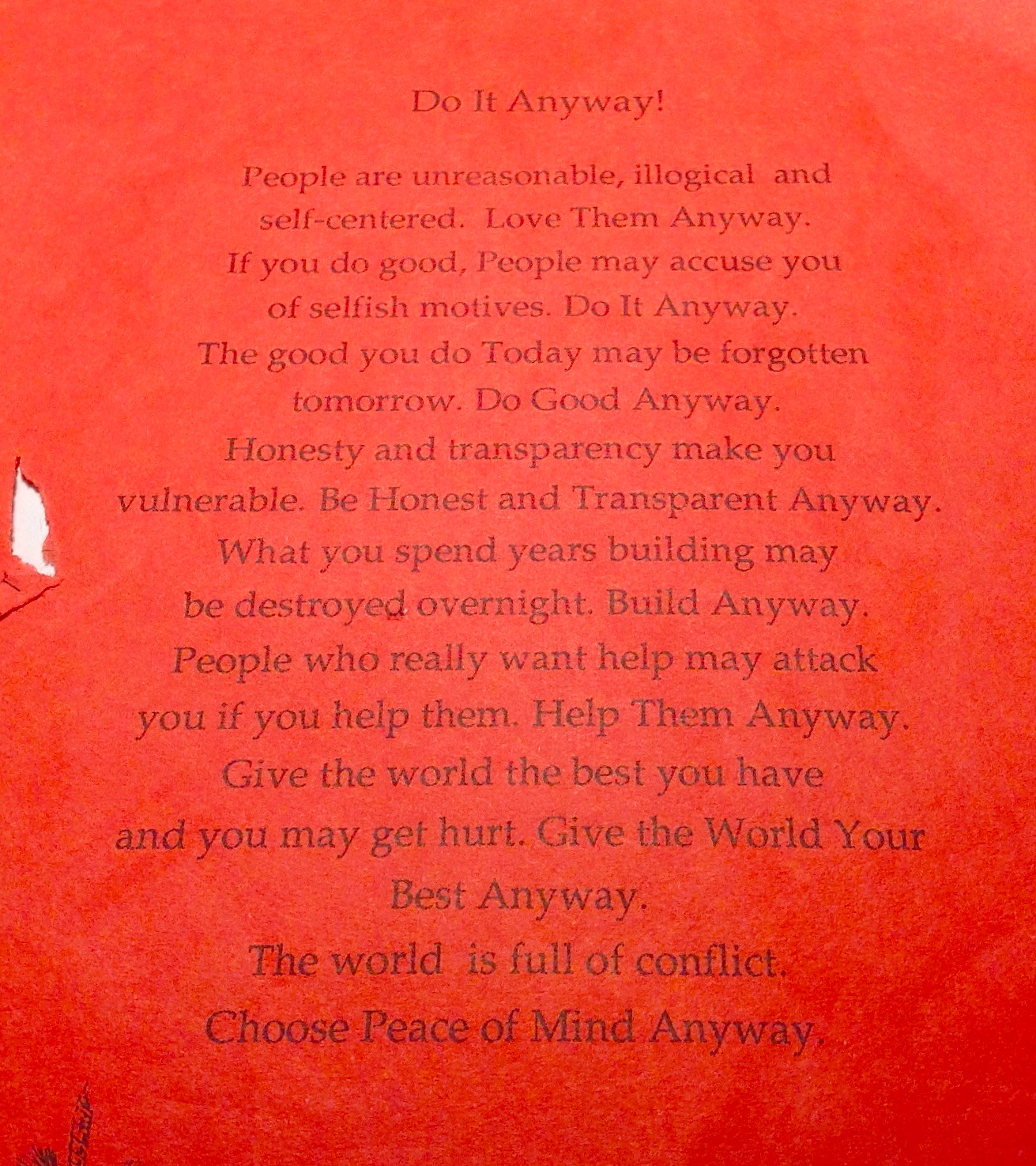The image is a color photograph of a vivid red piece of construction paper, slightly faded in the middle with a rip on the left-hand side. The gray text on this paper, though faint, conveys an inspirational message titled "Do it anyway!" It begins with: "People are unreasonable, illogical, and self-centered. Love them anyway. If you do good, people may accuse you of selfish motives. Do it anyway. The good you do today may be forgotten tomorrow. Do good anyway. Honesty and transparency make you vulnerable. Be honest and transparent anyway. What you spend years building may be destroyed overnight. Build anyway. People who really want help may attack you if you help them. Help them anyway. Give the world the best you have and you may get hurt. Give the world your best anyway. The world is full of conflict. Choose peace of mind anyway." This poignant piece serves as a reminder to persist in positivity and integrity despite the challenges and adversities faced.